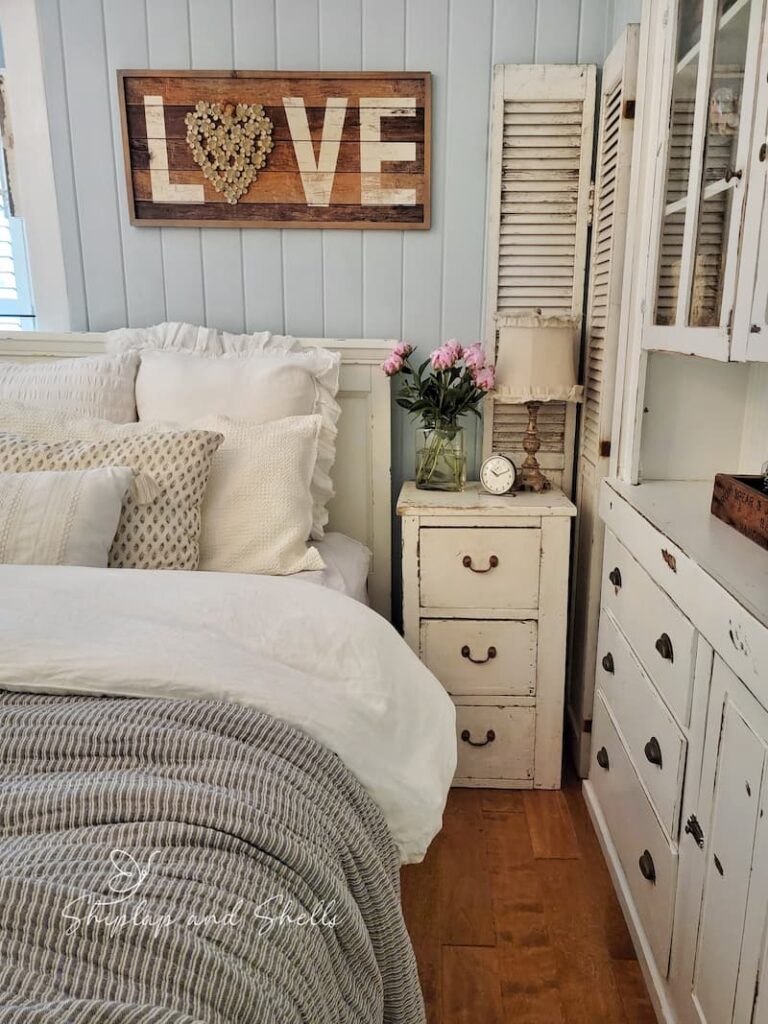This photograph captures a vintage chic bedroom with a predominantly wooden and antique aesthetic. The centerpiece of the room is a bed adorned with numerous pillows in white, gray, and cream, set against a white headrest. The bedding features a mix of a black and gray vertically striped comforter and a gray throw blanket with a straight pattern. Above the bed, a decorative wooden sign with the word "love" in white letters, where the 'O' is replaced by a heart, adds a personal touch against the white wall.

To the right of the bed stands an off-white nightstand, which hosts a vintage-style lamp, a clear vase filled with pink flowers, and a white clock. The floor consists of rich brown hardwood, contributing to the cozy ambience of the room. There's a set of old off-white shutters affixed to the wall, adding to the room's distressed look.

On the right side, there's an antique white dresser with visible blemishes and dark scuffs, enhancing its aged appearance. This dresser features an empty drawer space and cabinets with glass doors above it, blending storage functionality with decorative appeal. The room's style is completed by light blue rear walls that provide a soothing backdrop.

In the bottom left corner of the image, a watermark reading "Shplee and Shells" is visible, perhaps indicating the photo's origin or branding. The entire setting exudes a sense of comfort and timeless elegance, making it an inviting and thoughtfully designed space.